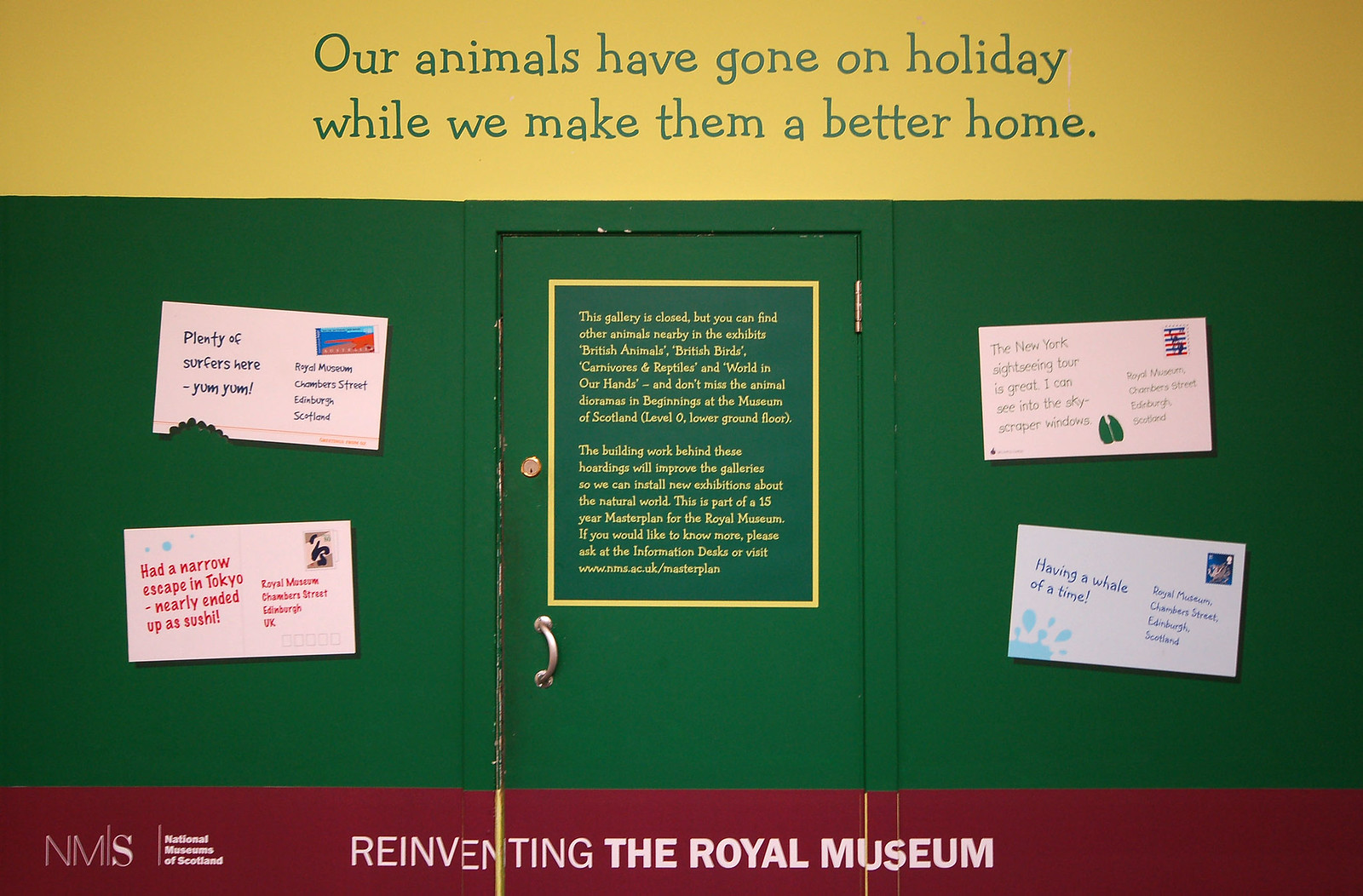The image depicts a green doorway set within a green wall, adorned with various announcements and postcards. At the top, a prominent gold banner reads: "Our animals have gone on holiday while we make them a better home." Below this, on the door, a sign informs visitors that "This gallery is closed, but you can find other animals nearby in the exhibits: British animals, British birds, carnivores and reptiles, and world in our hands. And don't miss the animal dioramas in Beginnings at the Museum of Scotland, level 0, lower ground floor." The door itself, complete with a handle and lock, suggests it is a real doorway leading to the closed gallery.

Surrounding the door are blown-up images of postcards, including one that reads, "The New York Sightseeing Tour is great. I can see into the skyscraper windows," while another humorously recounts, "Had a narrow escape in Tokyo, nearly ended up as sushi, sad end." Four posters are also scattered around the door.

At the bottom of the image, a maroon-colored bar boldly states, "Reinventing the Royal Museum," indicating ongoing renovations. Additionally, the logo "NMS" (National Museums of Scotland) appears at the bottom left, confirming the institution’s affiliation. Overall, the signage and accompanying materials suggest a thorough renovation effort to enhance the natural world exhibitions at the Royal Museum, part of a comprehensive 15-year master plan.